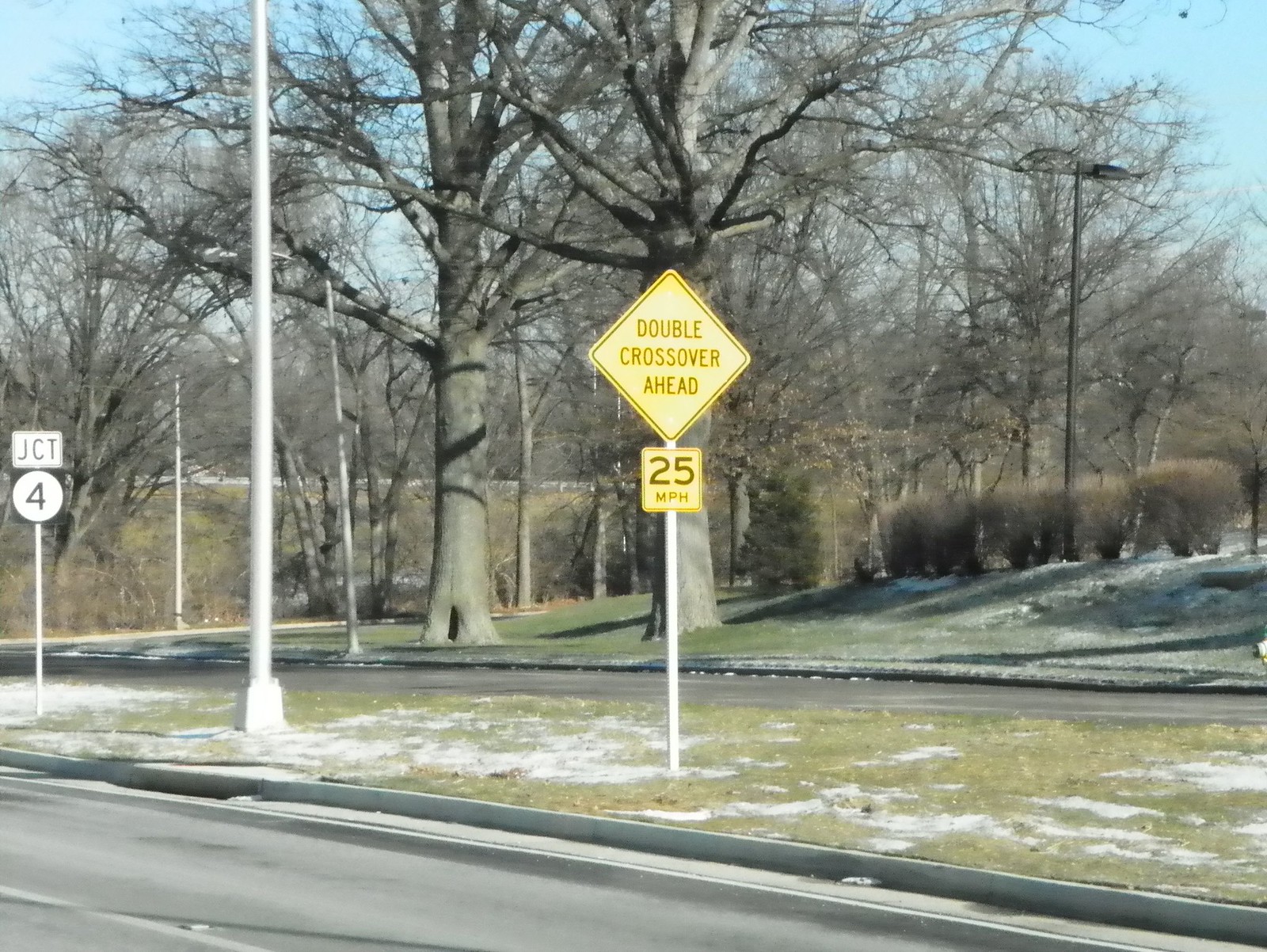This photograph captures a crisp, sunny day on a quiet street, marked by a glaringly blue sky devoid of clouds, hinting at cold weather suggested by a light dusting of snow on the ground. In the backdrop, tree-covered hills stretch into the distance, their clarity somewhat obscured by a thicket of leafless branches synonymous with late autumn or early winter.

On the right side of the frame stands a telephone pole or possibly a light pole, while the left side features another pole protruding upwards, which remains ambiguous in function but adds to the street’s character. Dominating the center are two large, barren trees, standing prominently on a grassy median that divides two roadways. Centrally positioned on this median is a yellow traffic sign emblazoned with the warning, "Double Crossover Ahead," stationed atop a white pole. Beneath this, another yellow sign clearly states a speed limit of "25 MPH" in black letters.

To the left of this main sign, a tall white or silver pole extends vertically, towering beyond the photograph’s upper limit. Adjacent to it, a smaller pole holds a rectangular sign reading "JCT" in black letters, with a circular white sign bearing the number "4" right below it. This meticulously detailed scene encapsulates a serene yet structured street landscape bathed in wintry sunlight.